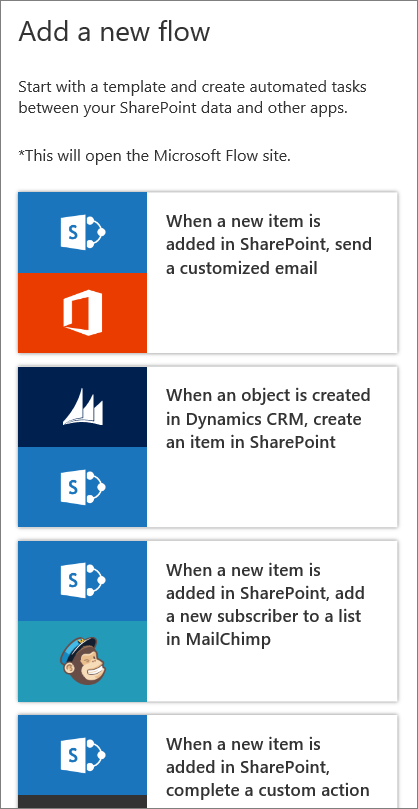In this image, we see the 'Add a New Flow' section of what appears to be a website manager application, possibly related to Microsoft Flow. The interface features a clean, white background bordered by a thin black line. At the very top of the section, 'Add a New Flow' is prominently displayed in bold black letters. Beneath this heading, the text explains: "Start with a template and create automated tasks between your SharePoint data and other apps. This will open the Microsoft Flow site."

To the left side of the section, several logos are displayed, indicating different services and applications that can be integrated. To the right, there is descriptive black text outlining various automation templates available:

1. "When a new item is added in SharePoint, send a customized email."
2. "When an object is created in Dynamics CRM, create an item in SharePoint."
3. "When a new item is added in SharePoint, add a new subscriber to a list in MailChimp."
4. "When a new item is added in SharePoint, complete a custom action."

The image portrays a clear and organized interface designed to facilitate the setup of automated workflows between various applications and SharePoint.